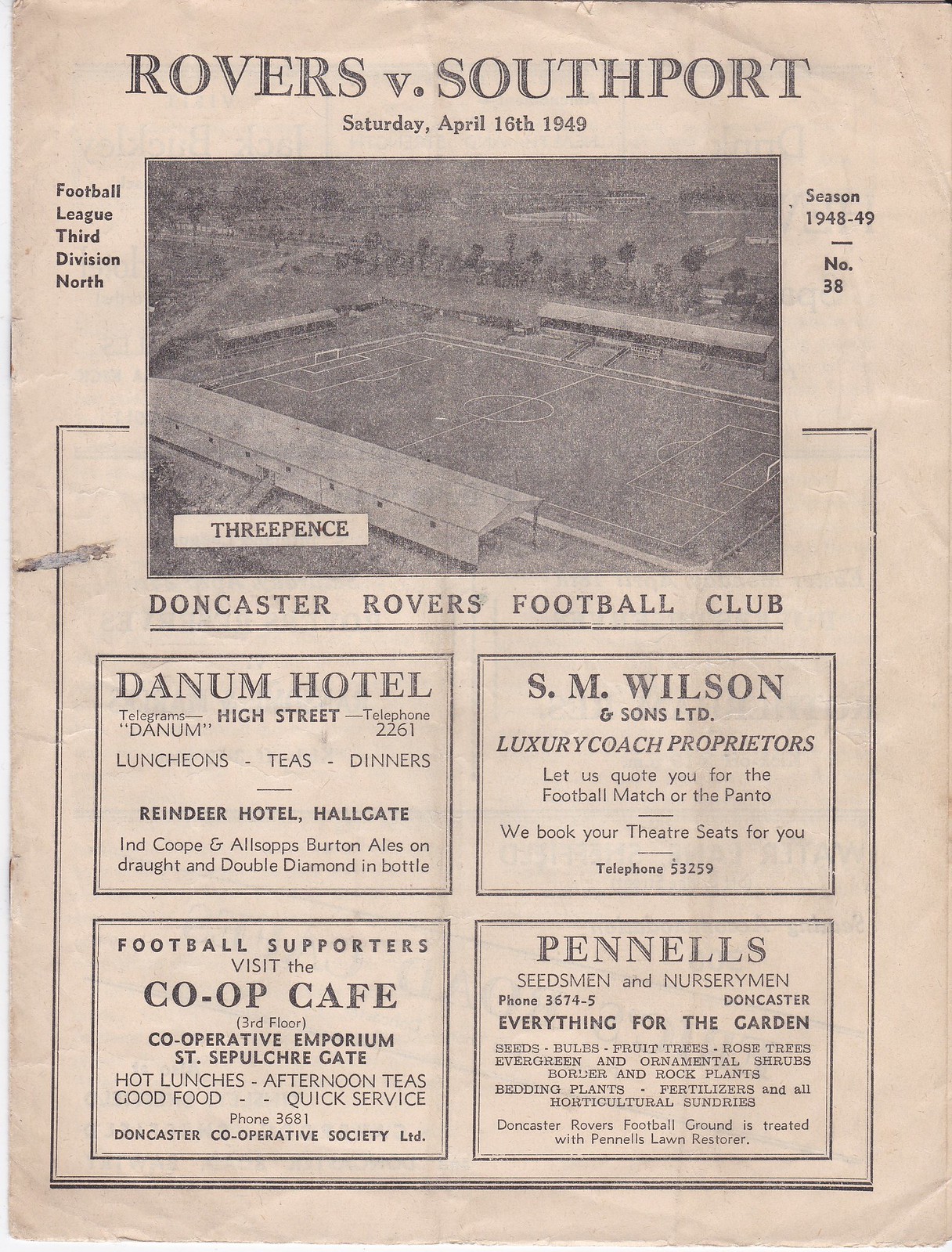The image depicts an old newspaper snippet or sports program cover from April 16, 1949, showcasing a match between Doncaster Rovers and Southport. The program, marked by yellowed paper and worn edges with a large scuff mark on the left, prominently displays "Rovers vs. Southport" in black letters at the top. Below the heading, it indicates the match date and features a black and white, somewhat faded, aerial photograph of an empty football stadium. The left side reads "Football League 3rd Division North" and the right side notes "season 1948-49, number 38." Underneath the photo, it states "Doncaster Rovers Football Club." The lower part of the program contains four rectangular advertisements for the match sponsors: Danum Hotel on High Street, S.M. Wilson Luxury Coach Proprietors, Football Supporters Visit the Co-op Cafe at the Cooperative Emporium St. Sepulchre Gate, and Pennell's Seedsmen and Nurserymen promoting "Everything for the Garden." The detailed advertisements include addresses and phone numbers, and the overall design, with its pink-tinted and black-and-white background, evokes a strong sense of historical charm.